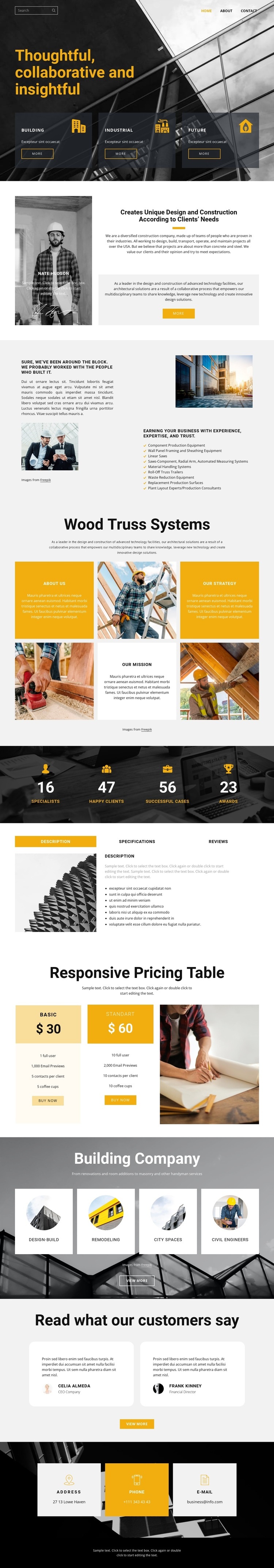The website has a skewed layout, making images appear wider than they are tall. At the top of the homepage, there are navigation links labeled "Home," "About," and "Contact." The site uses terms like "thoughtful," "collaborative," and "insightful" to describe its mission. There is a button labeled "More," which leads to sections titled "Industrial," "Future," and other categories, but much of the accompanying text appears to be placeholder content typical of a template.

Following this section, the site features a statement: "Create unique designs and construction according to client needs." It provides a detailed company description, emphasizing a diverse team with proven industry expertise. The company prides itself on designing, building, transporting, operating, and maintaining projects across the USA, while valuing client opinions and aiming to meet their expectations. However, despite this extensive information, the specific name of the website or company remains unclear in the provided content.